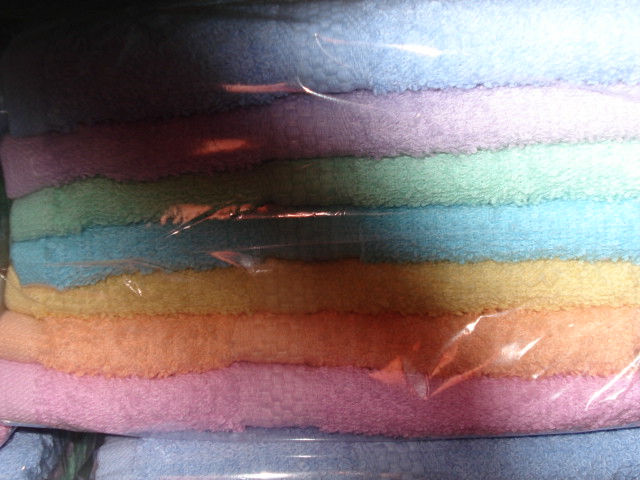This is a detailed, close-up photograph of high-quality, pastel-colored bath towels, meticulously folded and still encased in their original plastic packaging, likely on display on a shelf. The towels, made from terrycloth with a beautiful nap and textured borders just above the tightly woven selvedge, showcase a harmonious range of colors including pink, burnt orange, seafoam green, seafoam blue, pastel blue, pastel green, purple, yellow, and orange. Arranged in a crisscross pattern with one package laid horizontally across two others, the stack of approximately seven towels captured with a reflective sheen from the plastic wrap also demonstrates a slight shadow in the image's center, indicating the use of a flash during the photograph. The careful folding and plastic enclosure highlight their pristine, ready-for-purchase condition.